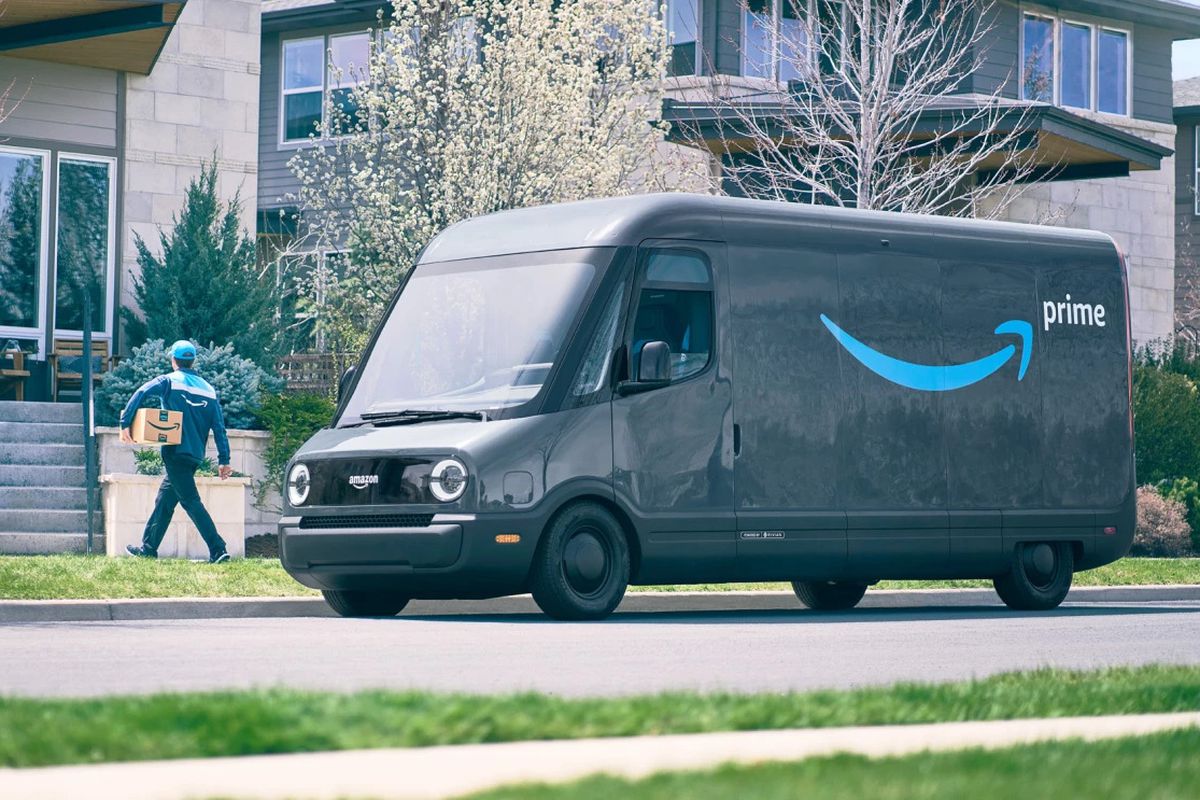A photo captures an Amazon Prime delivery truck parked on a residential road. The vehicle, resembling a rectangular van with basic black tires, is adorned with a prominent dark gray exterior, a blue arrow, and a white "Prime" logo. It is positioned next to a large, upscale house. To the left of the image, the delivery driver can be seen holding an Amazon package in his left arm as he walks toward the house's concrete staircase. The setting suggests the routine yet vital task of delivering packages to customers.